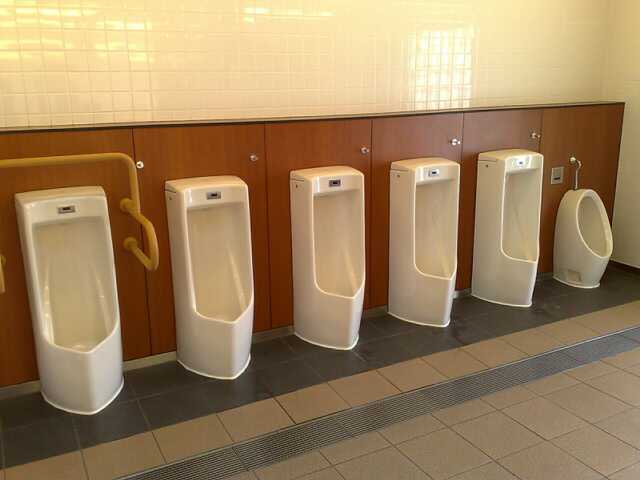This is a color photograph of a men's bathroom, captured in a horizontal rectangular frame. Six urinals, seemingly made of white porcelain, are installed against the back wall in a diagonal formation from the lower left corner toward the center-right. The wall they are mounted on has a distinct division: the upper part is covered in shiny white tiles, while the lower section features dark brown or black cabinetry with metal locks.

Five of the urinals are tall and rectangular, each equipped with a horizontal metal flush switch at the top center. The bowl of these urinals has an angular, pointed design. The sixth urinal, positioned at the far right, is notably smaller and circular, likely intended for children. This smaller urinal is positioned lower down, and to its left, on the wall, there's a small silver panel.

A noticeable yellow grab bar is placed above and next to the far-left urinal, suggesting accessibility considerations. The wall behind the urinals is covered with either yellow or cream tiny tiles, while the floor features a combination of blue and white tiles, interspersed with brown and black tiles. Additionally, there is a decorative strip running through the middle of the floor tiles and a grating near the urinals likely intended for drainage.